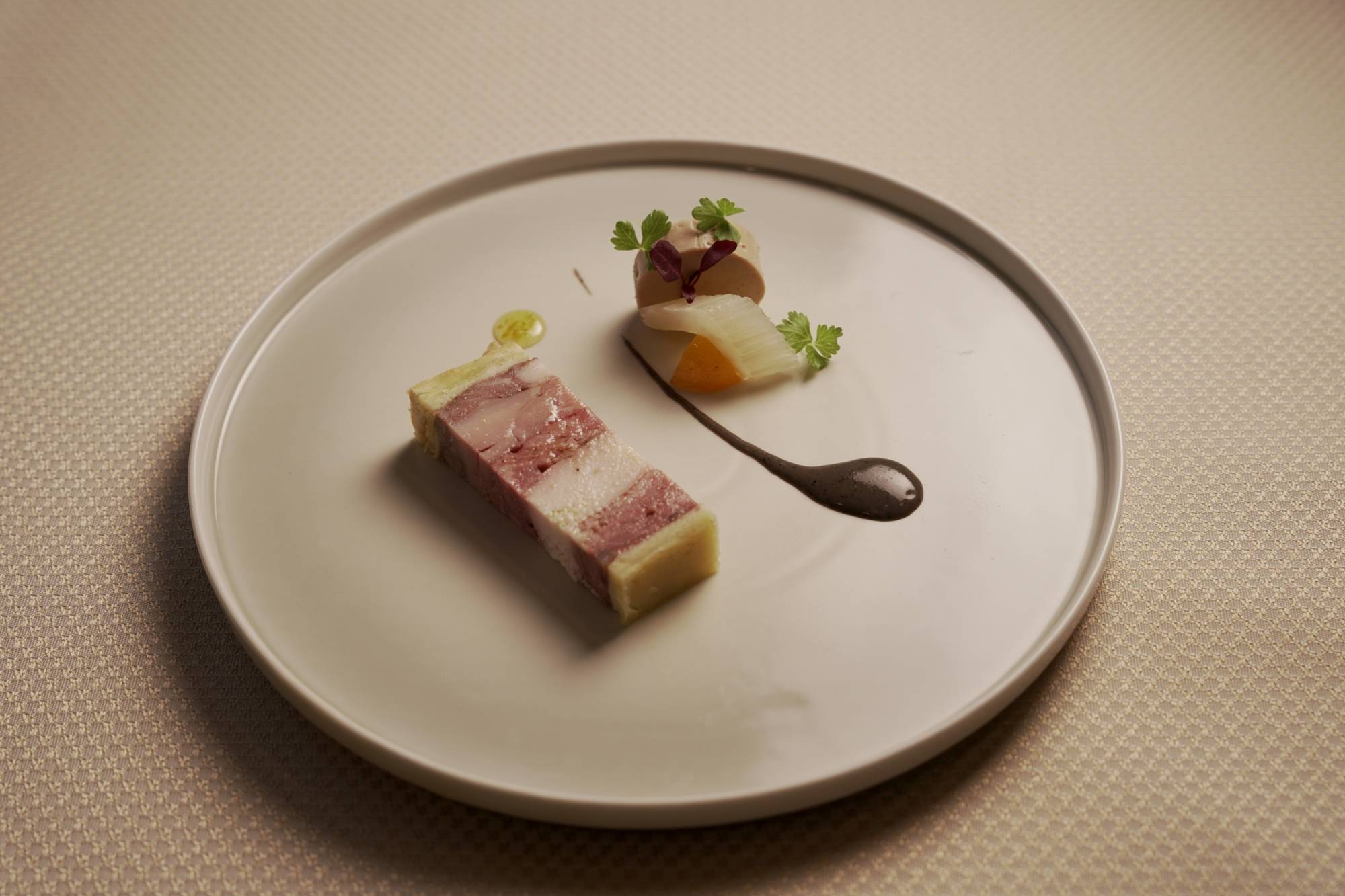The image features a gourmet meal artfully arranged on a modern, gray circular plate with a distinctive hard edge, set against a beige or checkered background. At the center of the plate lies a small, rectangular serving that appears to be layered, resembling a lasagna, with pinkish-brown shades and white layers. To the left is a dark-colored sauce, perhaps chocolate, artfully applied in a teardrop shape. On the right side, a garnish of vibrant vegetables, including something orange and small greens, adds a splash of color. The presentation is minimalist and stylish, suggesting an upscale appetizer or dessert, characterized by a careful, contemporary plating design.